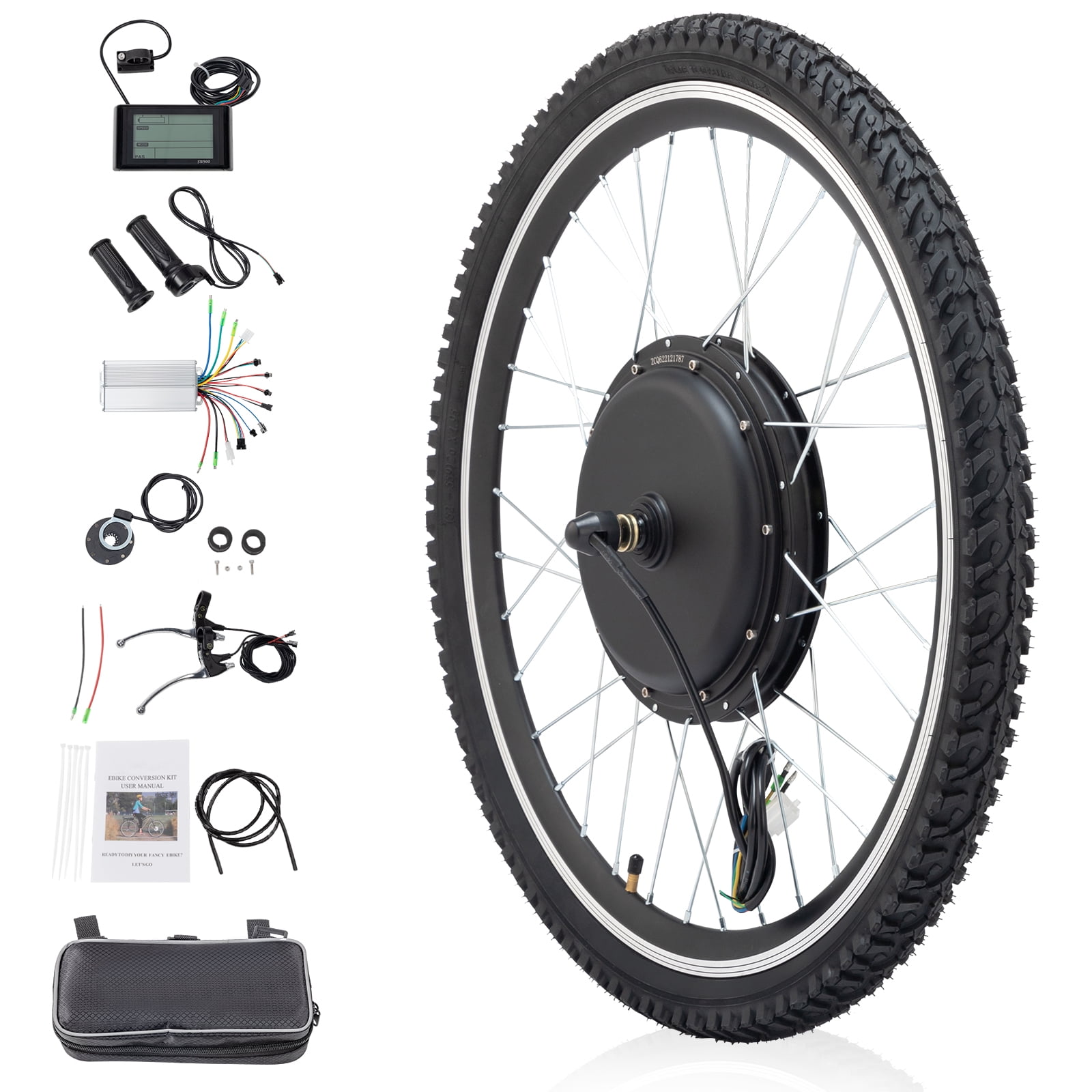The image depicts a comprehensive bicycle wheel conversion kit. The central and most prominent aspect on the right is a black bicycle tire with a silver rim, featuring a yellow air valve and equipped with silver spokes. Notably, a coiled black electrical cord protrudes from the hub, suggesting it contains electronic components. On the left side of the image, a series of smaller pictures illustrate various parts included in the kit. At the top is a digital monitor with black cables connected to it. Below the monitor are two hand grips, one of which is equipped with a cord, while the other is a standard rubber grip. Next is a white control box with a multitude of colorful wires (green, red, yellow, black, white) extending from it. This section also pictures four small coils of black wire, assorted hardware including hub adapters, and components with splice connectors. Further down, the images show more coiled wires in red and black, an instruction manual, zip ties, and a black zippered rectangular case, resembling a fanny pack. This detailed photo provides a clear view of a bicycle wheel charging kit conversion, complete with all necessary accessories for assembly and installation.